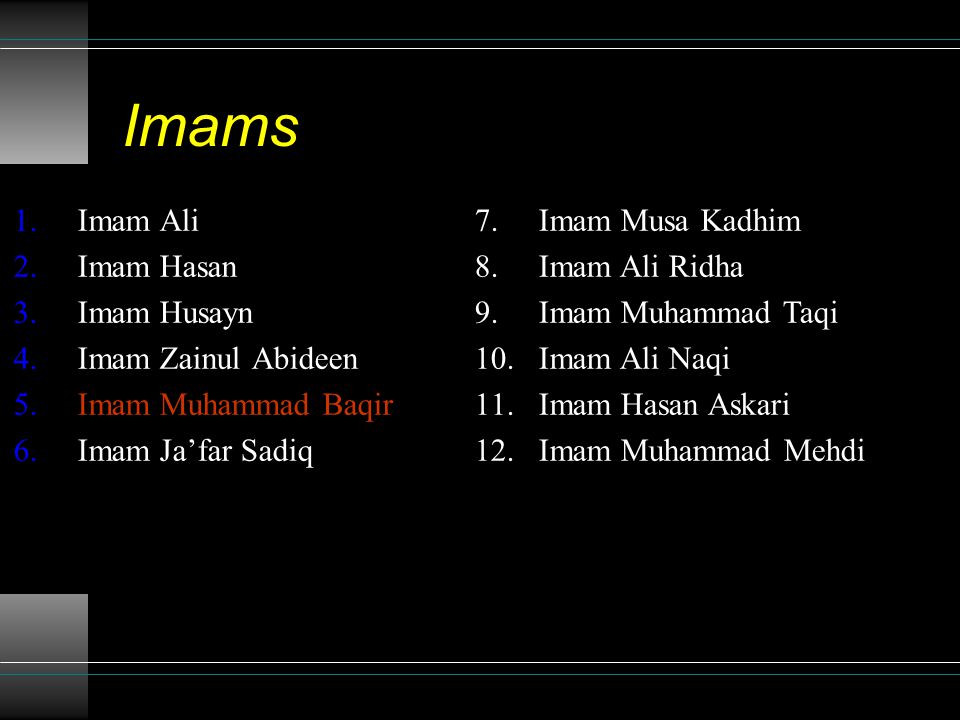The image is a detailed PowerPoint slide with a black background, featuring the title "Imams" in yellow italics at the top left corner. There are twelve phrases listed below it in two columns, each accompanied by numbers in blue for the left column and white for the right column. The left column, numbered one through six, includes: 1. Aymar Ali, 2. Aymar Hasan, 3. Aymar Kuzenya, 4. Aymar Sadu Abedin, 5. Aymar Muhammad Baku (highlighted in red), and 6. Aymar Jafar Sadiq. The right column, numbered seven through twelve, lists: 7. Aymar Buzar Qardin, 8. Aymar Ali Rida, 9. Aymar Mahad Daki, 10. Aymar Ali Labki, 11. Aymar Hasan Azkari, and 12. Aymar Mahad Muhammad Madi. The slide also features thin white and light blue lines at the bottom and a thin white line across the top, adding a structured aesthetic to the presentation.